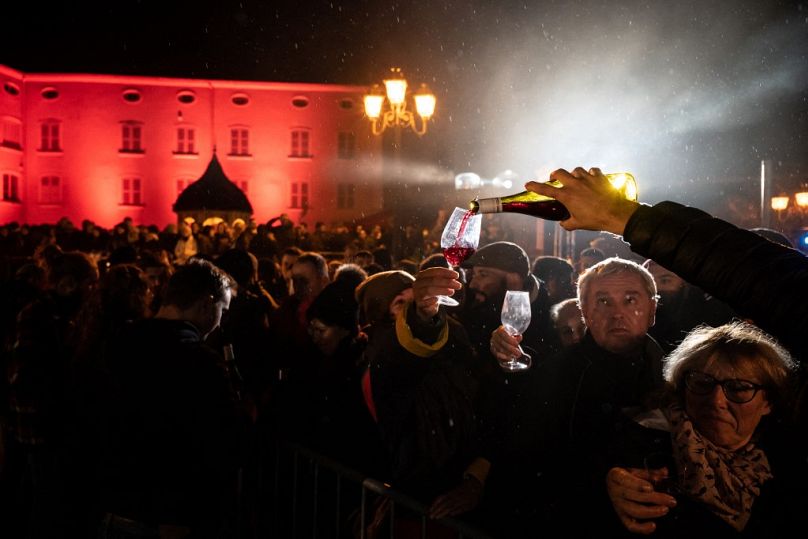This nighttime photo captures the vibrant atmosphere of an outdoor festival or celebration. A large crowd fills the street, with many attendees holding up glasses as an unseen hand from the right side of the image pours red wine into them. In the center of the scene, a tall lamppost with four lights illuminates the gathering. To the left, a grand building, bathed in red light, serves as a dramatic backdrop to the festivities. The expressions of the people in the crowd seem varied and open to interpretation, adding to the captivating and enigmatic nature of the image.